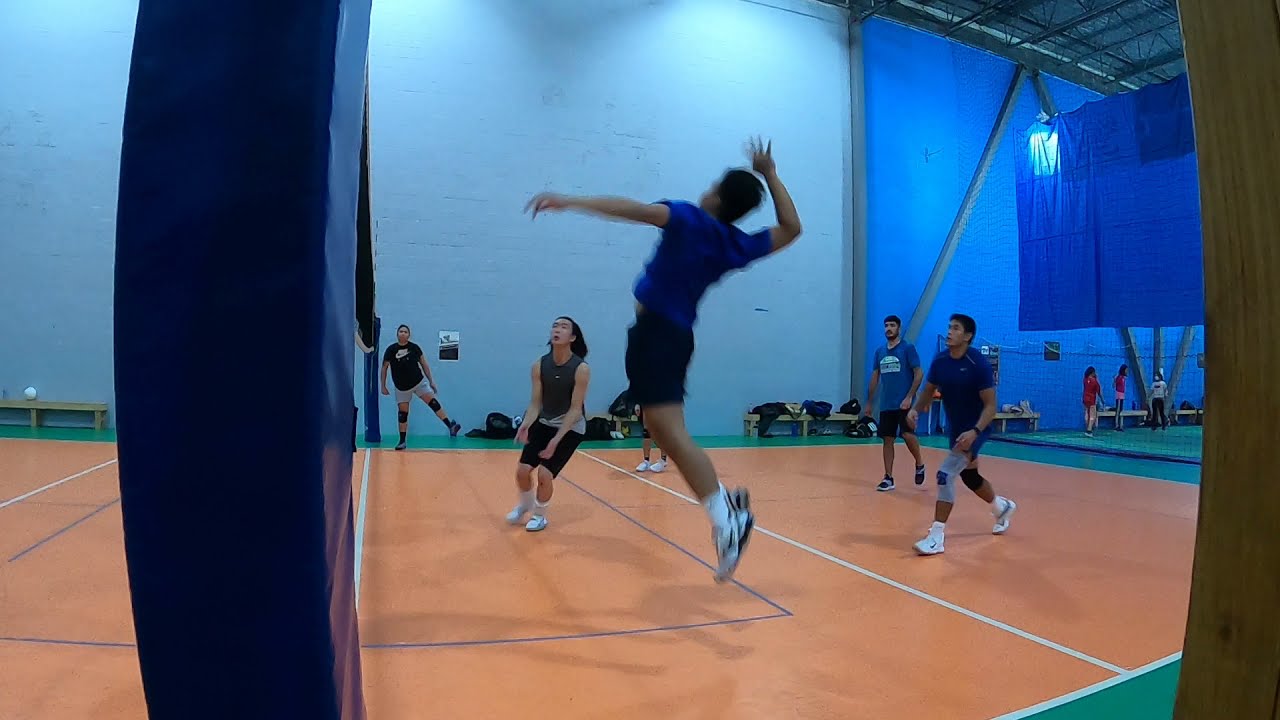The photo captures a dynamic moment of an indoor volleyball game, focusing on one side of the court, taken from midcourt off to the side. It prominently features a player, likely the ace, on the left side of the image who is in mid-jump with his right arm drawn back, ready to spike the ball that hovers above him. The setter, positioned centrally, appears to have just executed a bump set, as indicated by the relaxed position of his arms. Surrounding them, the team's right hitter is positioned wide, while the three back row players are poised and anticipating the next move.

The setting is a spacious, high-ceilinged gymnasium with largely undecorated walls. The court has a smooth brown surface with green accents on the outer edges. The image is devoid of any text and contains a range of colors including light blue, brown, green, pink, orange, dark blue, black, and red. The volleyball net appears towards the left, though it visually resembles more of a purple post due to the photo's angle.

There are additional people visible in the background, partially caught in the frame, enhancing the sense of a lively tournament taking place. The overall scene conveys the intense focus and anticipation of the players as they engage in this critical moment of the match.